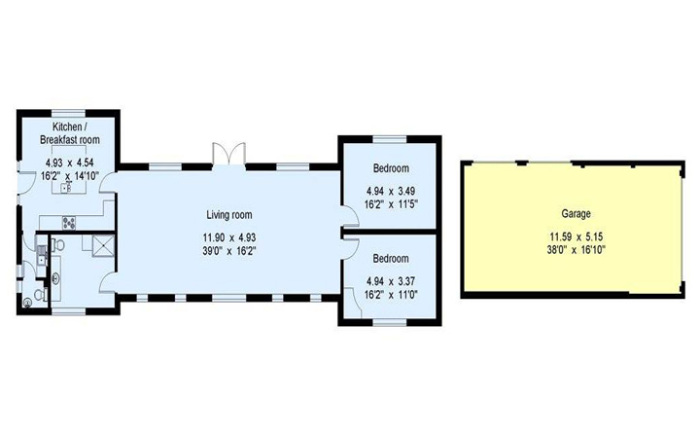In the photograph, we are examining a detailed floor plan. The plan includes a garage, highlighted in yellow, with dimensions clearly marked in black text. The garage measures 11 feet by 11.59 feet by 5.15 feet, and below these measurements, an additional size of 38 feet by 16.10 feet is indicated.

The floor plan also displays the layout of an apartment, highlighted in blue, within a large rectangular space. The apartment comprises two small bedrooms, a living room, a kitchen, and a bathroom. Both bedrooms have similar dimensions and feature two door entryways each. The living room, with its dimensions marked, sits centrally within the layout.

The main entrance to the apartment leads directly into the living room. To the left of the entrance, there is a doorway to the single bathroom in the apartment. Adjacent to the bathroom, you will find the kitchen and breakfast area, which includes a door leading outside. This area also appears to have a window, providing additional natural light. Overall, this floor plan provides a comprehensive view of the apartment’s layout and dimensions.